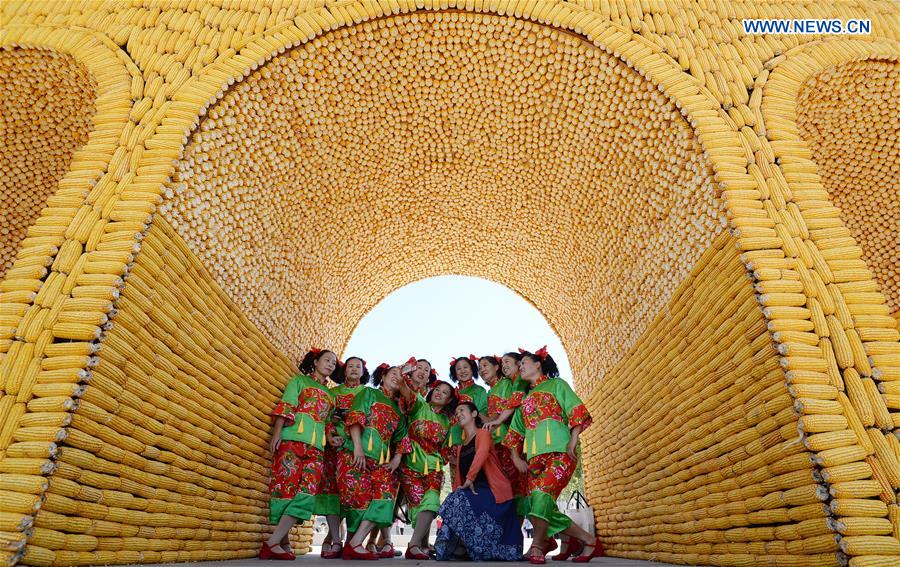This is a color photograph, likely from a news source (www.news.cn visible in the upper right corner), depicting a group of approximately ten young Asian women, possibly part of a dance troupe, standing underneath a massive archway constructed entirely of corn cobs. The women all wear identical uniforms consisting of red shorts or pants with green trim, black shirts with red across the chest, and three yellow tassels hanging from their bodices. They complete their outfits with red Mary Jane-style shoes and red ribbons tying their hair back into pigtails. Central to the group is a woman in a coral-colored coat over a blue dress, who is kneeling and placing one hand on her knee. Another woman appears to be holding a phone, perhaps to take a selfie. The corn cob archway, which has several sections and forms a tunnel-like structure, features corn cobs arranged to show their sides on the walls and pointing down from the top. The image captures the women standing closely together under this elaborate and textured archway, with parts of the sky visible in the background.